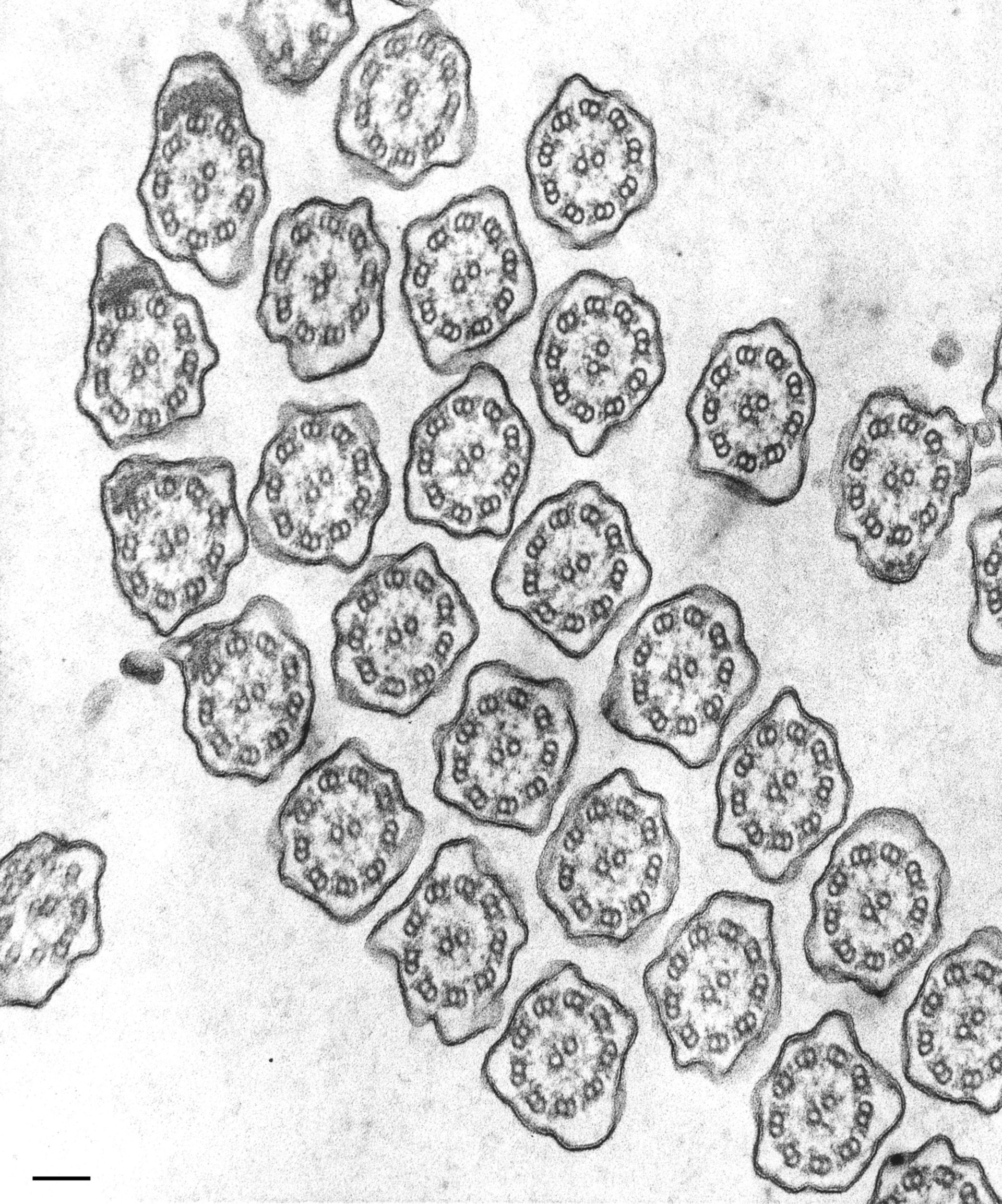The large, vertical, rectangular image appears to be an intricate drawing rather than a photograph. The background is primarily light gray with textured darker areas, resembling cloth more than paper. The illustration depicts numerous irregularly shaped objects, each with a circular design composed of smaller circles, and featuring a central pair of circles. These objects, which could be cells or some other microscopic life forms, are dispersed unevenly across the image. The entire scene is rendered in black and white, and the blobs have a jelly-like appearance with penciled outlines. The background appears smeared, giving it a dirty, rubbed effect, consistent with pencil shading. The detailed, repeating circular patterns within each blob enhance the impression of a microscopic view, possibly digitally enhanced to highlight the intricate details.